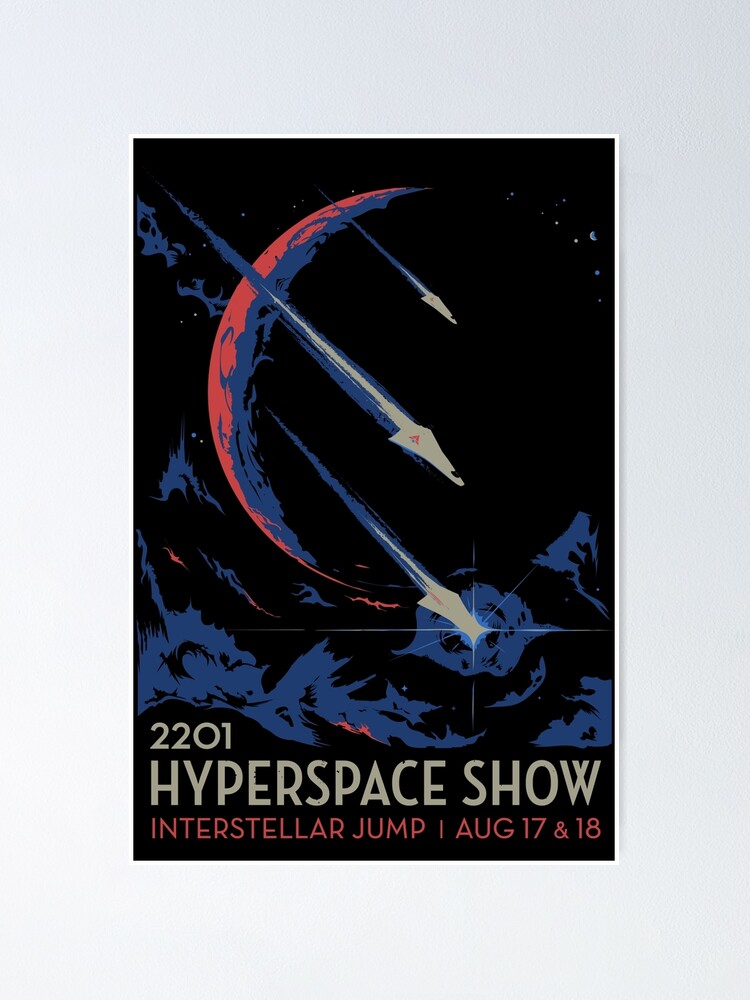The detailed poster image advertises a fictional event titled "2201 Hyperspace Show: Interstellar Jump," scheduled for August 17th and 18th. The central graphic depicts three sleek spacecraft zooming across the foreground of a shadowed planet, leaving dynamic air trails behind them, giving an impression of rapid movement through space. The spacecraft, rendered in white with red and blue logos, seem to pierce through the dark, space-themed backdrop filled with hints of bluish space debris or gases.

The background planet is primarily black and shadowed, accented by subtle red and blue tints at its edges, almost indicating a new moon phase. The entire composition rests on a gray background with a double matting, the outer one blue-gray and the inner one white, adding depth to the presentation. Text details include "2201" at the top, "Hyperspace Show" below it, and "Interstellar Jump: August 17th and 18th" at the bottom, with crucial dates and event specifics highlighted in red for emphasis. This artful blend of dark hues and strategic color highlights creates a futuristic, high-speed scene that emphasizes both the advanced technology of the ships and the expansive, mysterious backdrop of space.